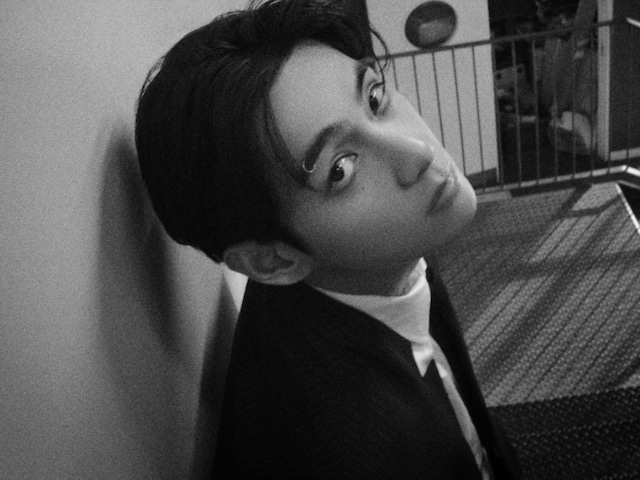This black and white photo captures a young Asian man with a serious expression, looking up diagonally into the camera. His head is tilted slightly to the right. He has black hair parted in the middle, falling close to his ears, and he’s adorned with a small hoop piercing in his right eyebrow. He wears a white turtleneck paired with a black blazer, giving him a stylish, contemporary appearance reminiscent of a Korean pop star. The photo, seemingly modern but presented in black and white, shows him leaning against a wall near a metal railing and a set of stairs. In the blurred background, there's an open door revealing indistinct items. He is posing, but his expression remains serious as he makes eye contact with the camera from below.